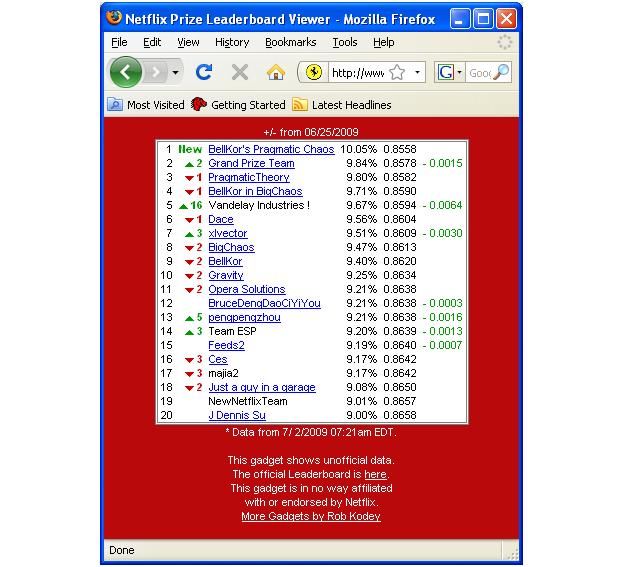The image is a detailed screenshot of a web page viewed in Mozilla Firefox, evident by the Mozilla Firefox logo on the blue header at the top. The web page is titled "Netflix Prize Leaderboard Viewer" and has standard browser elements such as the minimize, maximize, and close buttons. In a light gray header beneath the blue one, there are usual navigation menus: File, Edit, View, History, Bookmarks, Tools, and Help.

Below this, the browser's toolbar contains a green back button, a gray forward button, a blue refresh button, a gray X to stop loading, and a home button, followed by a URL bar starting with "http://www". Next to this is another search bar, formatted for Google. The bookmarks toolbar below this lists "Most Visited," "Getting Started," and "Latest Headlines."

The main content of the page is focused on the Netflix Prize Leaderboard, spanning from 2005-2009. This leaderboard, displayed against a red background, ranks various participants with precise metrics. For example, the top entry is “Bellcore's Pragmatic Chaos” with a score of 10.05% and an RMSE (Root Mean Squared Error) of 0.8558. The leaderboard continues down to the 20th ranking, which is for “J. Dennis Hsu” with a score of 9% and an RMSE of 0.8658.

At the bottom of the leaderboard, there are disclaimers stating, “This gadget shows unofficial data” and “This gadget is in no way affiliated with or endorsed by Netflix." There’s also a timestamp indicating the data is from July 2009 at 7:21 Eastern Time, and credit is given to the creator, Rob Coray.